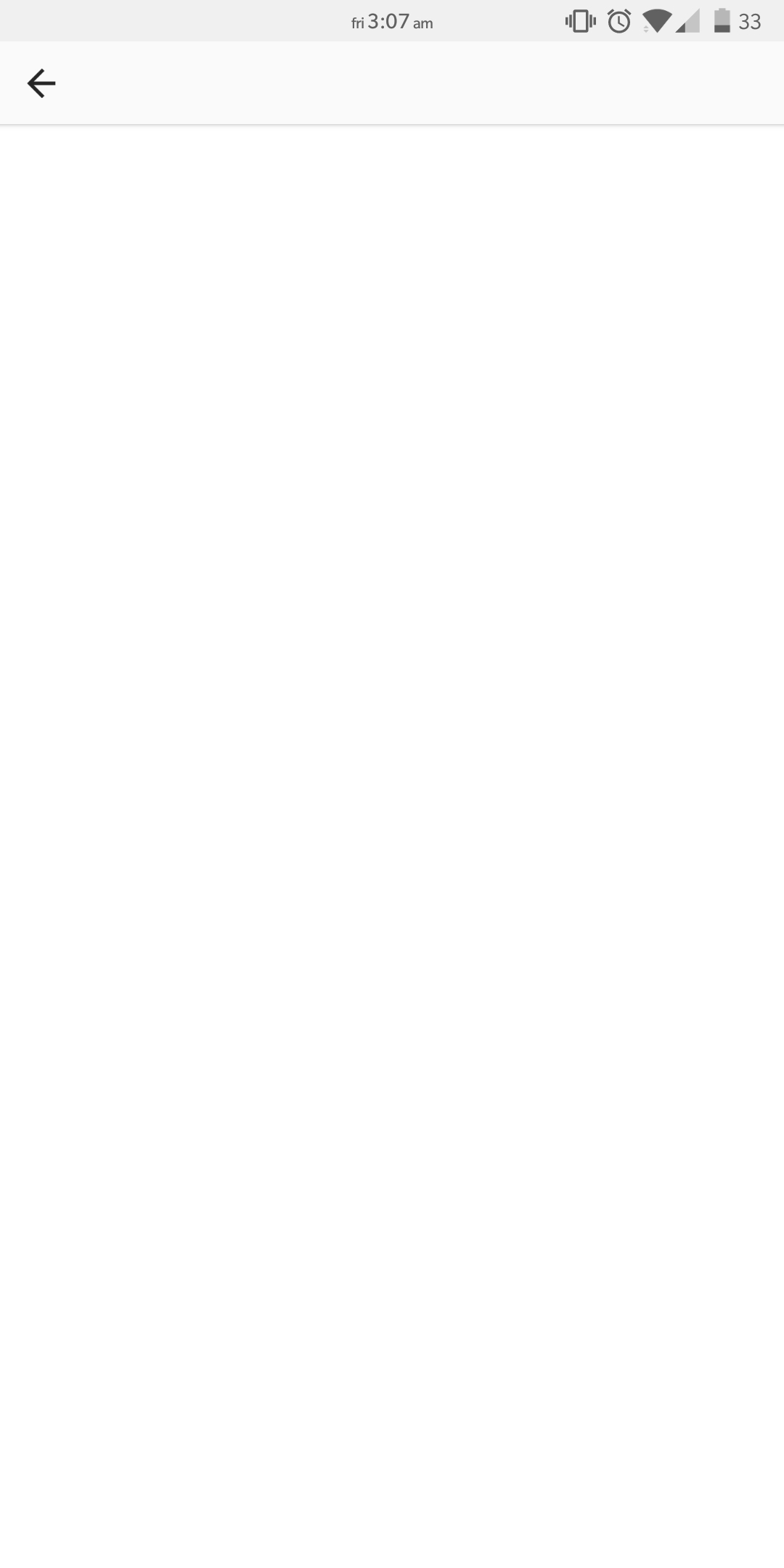The image depicts the upper portion of a smartphone's screen against a completely white background with no visible borders. The display is divided into two main sections. The top section features a gray banner, slightly darker than the lower area. At the center of this gray banner, the time is displayed in small characters: "FRI" indicating Friday, followed by "3:07 AM."

To the right of the time, several icons are present. The first is a toggle icon resembling a phone with two lines on each side. Next to it is a clock icon, showing two hands and two small lines at the top representing bells. Further to the right, there is a fully filled Wi-Fi icon and a partially full signal strength icon. Next to the signal icon, the number "33" is displayed, and beneath it, on the left side, is a left-pointing arrow. The entire gray banner is otherwise empty, providing a simple and clean interface.